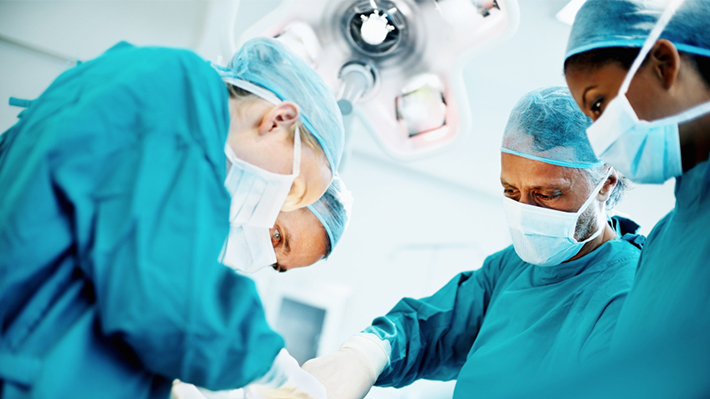In this image, taken from a low, upward-facing angle, we see four surgeons deeply focused on their work, likely operating on a patient. They are all dressed in aqua or blue-green scrubs, complemented by white gloves and light blue masks. Each wears a matching blue hairnet, which maintains the sterile environment of the operating room. The surgeons' hands converge towards a central point, probably an operating table. The room is pristine and well-lit, with white walls and furniture, giving it a clean, clinical appearance. A prominent surgical light fixture, shaped like an X with various lights, is visible on the ceiling, which is also white. This overhead light adds to the brightness of the room. The image has a slight clockwise tilt, adding a dynamic perspective. Overall, the intense concentration of the surgeons and the organized, sterile surroundings suggest that this could be a stock photo capturing a moment in a high-tech surgical setting.